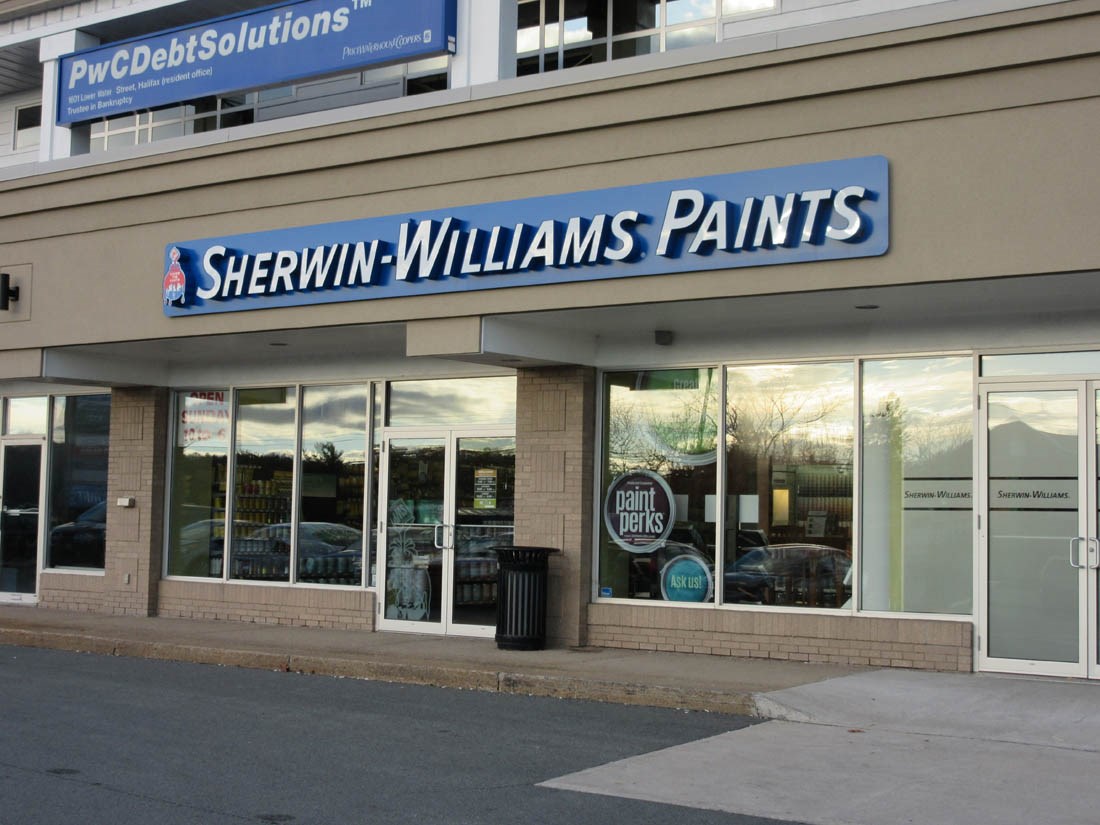A detailed and clean descriptive caption for the image could be:

"This image features the exterior of a Sherwin-Williams paint store. Prominently located near a road, the store's parking lot is visible in the foreground. The entrance is situated on the side of the building, flanked by a black trash can. Above the entrance, the Sherwin-Williams sign is prominently displayed, showcasing the iconic logo: a globe being covered by cascading paint in red, white, and blue hues. The text on the sign features 'Sherwin' with a notably larger 'S', and 'Williams' with a distinctively larger 'W', while the remaining letters in both words are uniformly capitalized but smaller in size. The store's glass windows reflect the vehicles parked outside, adding depth to the scene."